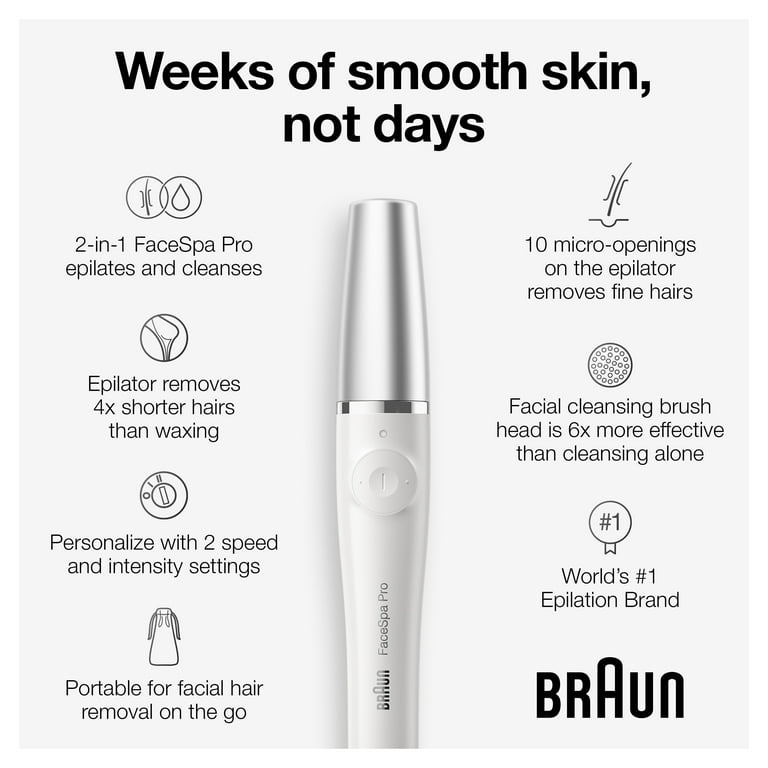This advertisement showcases the Braun FaceSpa Pro Epilator Pen against a light blue, silvery background. At the top, in bold black letters, it declares, "Weeks of smooth skin, not days." The ad highlights several key benefits of the product, including its dual functionality: it epilates and cleanses. One important feature mentioned is that the epilator can remove hairs that are four times shorter than those that waxing can remove. The text emphasizes the personalized settings, with two speed and intensity options, and its portability, ideal for on-the-go facial hair removal.

Furthermore, the epilator boasts 10 micro-openings designed to efficiently remove fine hairs, and the facial cleansing brush head is noted to be six times more effective than cleansing without it. The ad confidently claims Braun as the "world's number one epilation brand." In the lower-right corner, Braun's logo is prominently displayed in bold black letters, with the "A" noticeably elevated above the other letters in the brand name.